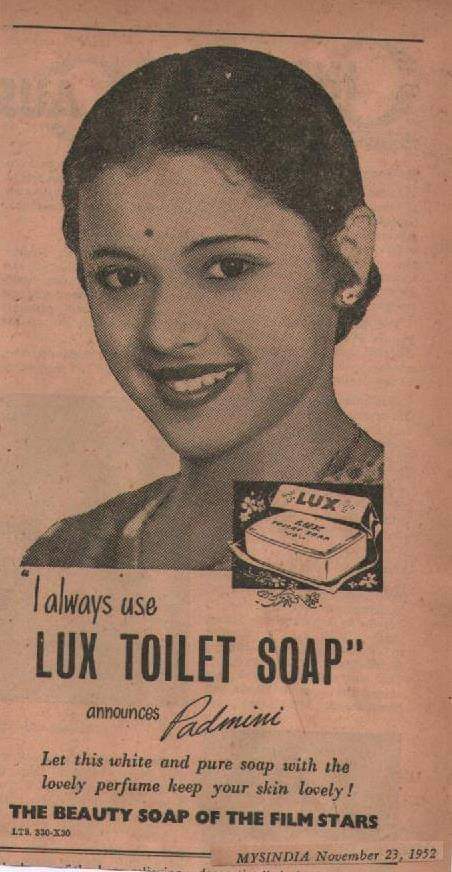This vintage 1952 advertisement for Lux Toilet Soap features an Indian woman with a traditional bindi on her forehead, suggesting her cultural heritage. Her hair is tied back, and her face shows a bright smile, rendered in a monochromatic sepia tone, giving the image a nostalgic and weathered appearance, as if it were from an old newspaper. Below her portrait is an illustration of the Lux soap bar. The text beneath her image is a quote that reads, "I always use Lux Toilet Soap," announced by Padmini, a renowned film star of the time. The advertisement further promises, "Let this white and pure soap with the lovely perfume keep your skin lovely." The layout presents a mix of script and sans-serif fonts, adding to the classic appeal and emphasizing the soap's association with beauty and glamour from the film world.